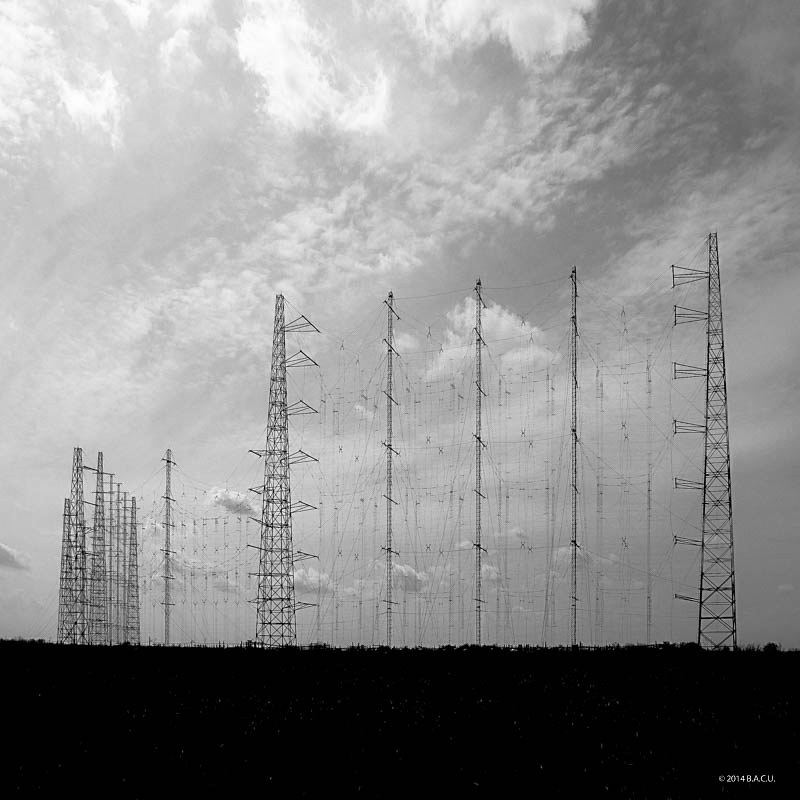This is a black-and-white photograph dominated by a striking sky filled with a mix of gray and white clouds. The horizon sits low, taking up just a fifth of the image, adorned with what appears to be a combination of grass, bushes, and tree tops creating a jagged line against the sky. Towering over this horizon are numerous steel electrical towers, drawing attention with their intricate lattice structures and vertical metal poles, all connected by a web of cables that span horizontally and vertically across the scene. On the left side, there is a noticeable cluster of smaller towers, adding to the complex network. At the bottom right corner of the photograph, the text "2014 BACU" is inscribed, indicating its copyright.